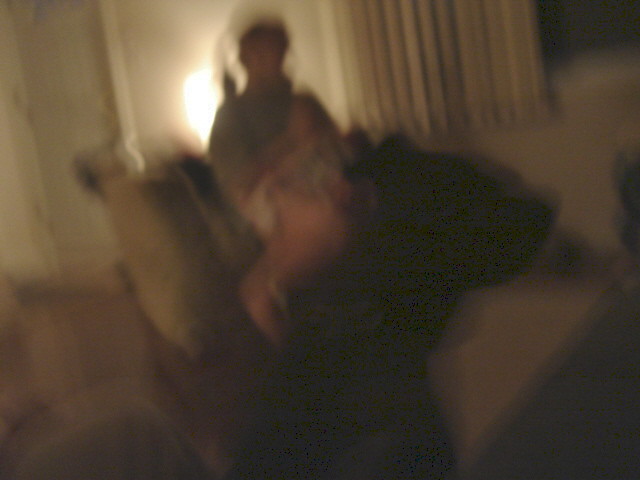In this image, captured inside a home, the photograph appears extremely blurry and distorted. On the left side, a white door is faintly visible, with a glowing light situated immediately to its right. In front of this light, the silhouette of a person is discernible, seemingly sitting in what could be a chair or a recliner. The chair's form is suggested but not clear due to the blurriness. To the right of the seated figure, partially open blinds reveal a dark window, contributing to the overall dim ambiance. The lower section of the photograph is predominantly dark, with a portion of the brown-colored floor being faintly visible on the left. The center of the image is dominated by a large, black area, possibly a shadow or uncertainty created by the poor image quality. This blend of elements results in a deeply obscured scene, challenging the viewer to piece together the home's interior context.